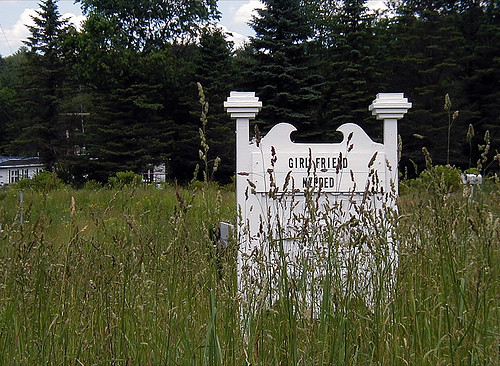This color photograph captures an outdoor scene bathed in uniform natural lighting. In the foreground, a field of tall grass sways gently. Dominating the scene is a white sign standing slightly right of center at the bottom of the image, anchored by two posts. The top part of the sign features an intricate design resembling two birds with curved beaks, facing each other. The sign, though slightly obscured by the tall grass, bears a bold, black inscription at the top that reads "Girlfriend needed." Beyond the sign, a line of darker-colored trees forms a natural backdrop. To the left of the image, closer to the horizon, rests a low white wooden building, adding an element of rustic charm to this idyllic landscape.